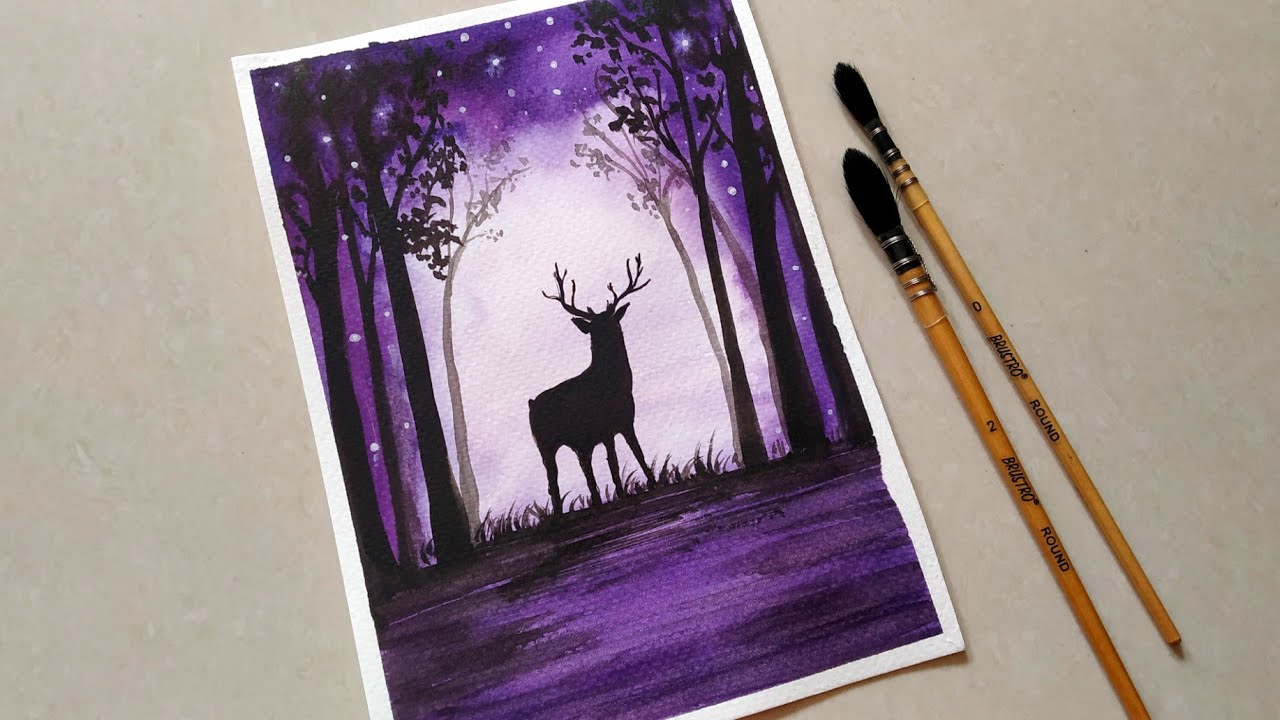This is a photograph of a textured piece of paper featuring a finished watercolor painting with a white border. The primary scene showcases a black silhouette of a deer with large antlers, standing in the middle of a forest. Flanking the deer are trees also rendered in black. The background is predominantly a mix of purple and black, with a smattering of tiny white dots representing stars against the purple sky. There is a bright white area behind the deer, possibly representing a moonlit or illuminated scene. Below the deer, the ground reflects the same purple and black hues. The entire image is laid at a slight angle with the top part tilted up and to the right. To the right side of this artwork, two narrow paintbrushes with black bristles and orange wooden handles are visible. They have writing on them in black, with the one on the furthest right labeled "brustro round 0" and the other labeled "brustro round 2." The background behind the sheet of paper is a subtle marbled light tan color.